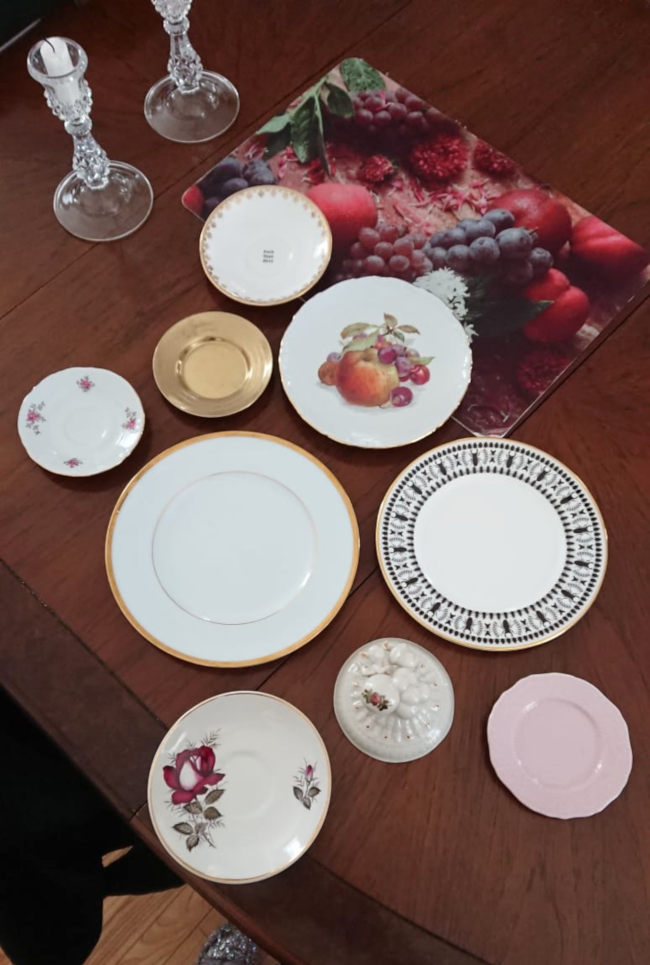The photograph depicts a top-down view of an ornate collection of decorative plates and tableware arranged on a dark reddish-brown wooden dining table. Scattered across the table are nine plates of varying sizes and intricate designs. Among them, one all-gold saucer stands out, while the rest are white with diverse decorative elements: a plate with a still-life painting of fruits (peaches, cherries, or apples), another with large painted red roses and stems, and others featuring floral motifs, scalloped edges, and ornate rims—including one with a blue repeating pattern.

In the upper left corner, there are two clear glass candlesticks holding short, burnt-down white candles, though only one candle is fully visible in the frame. At the center of the table is an item with enlarged close-up photographs of berries—possibly the back of a book or magazine, showcasing raspberries, cherries, strawberries, and blueberries. Also visible in the arrangement are a few pieces that suggest a rustic or culinary theme, such as what appears to be a placemat or a cutting board with a photographic design of fruit including peaches, grapes, and mint leaves, prominently placed in the upper right corner.

The entire setting gives an impression of an eclectic assembly of fine china and decorative tableware, more for display than for a coherent place setting, suggesting either an intentional artistic composition or a moment of transition in arranging the table.